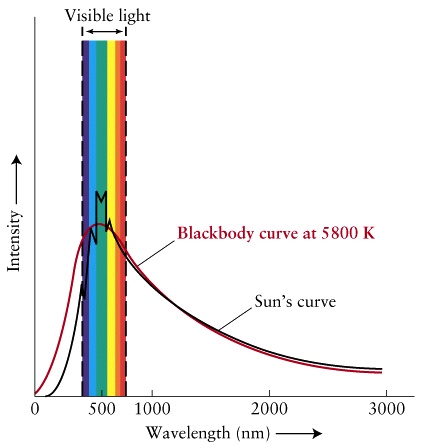The image is a detailed graph illustrating the relationship between wavelength and intensity. The x-axis, labeled "Wavelength (nm)," ranges from 0 to 3000, while the y-axis, labeled "Intensity," points upward. A prominent red curve, identified as the "Blackbody Curve at 5800K," stretches across the graph, starting near the top at the 500 nm mark and gradually descending towards the right, ending close to the 3000 nm point. This curve is distinctly marked in red font. Below this red line, a black line labeled "Sun's Curve" similarly slopes downward. At the 500 nm mark, vertical rainbow-colored bars indicate the "Visible Light" spectrum. The background of the graph is white, providing clear contrast for the colorful and labeled elements.